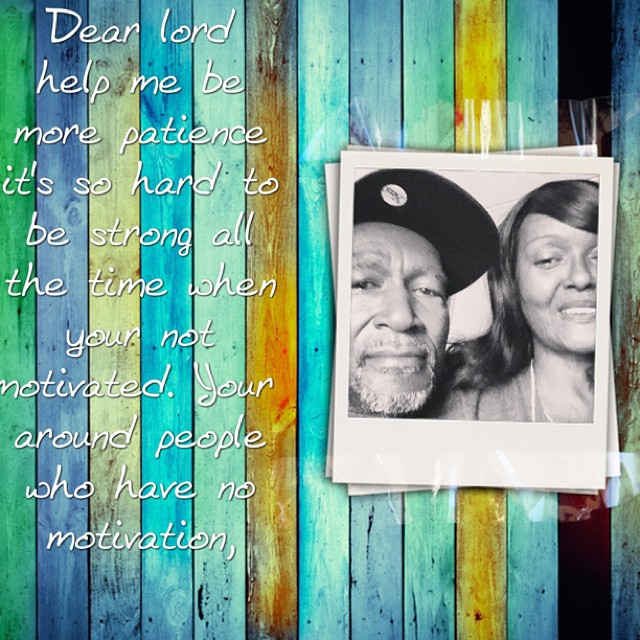This square image features an inspirational quote in white text on the left side that reads, "Dear Lord, help me be more patient. It's so hard to be strong all the time when you're not motivated. You're around people who have no motivation." To the right of the quote is a collection of Polaroid-style photographs of an older black couple, a smiling man with a baseball cap and goatee, and a woman with long hair swept to the side. The black-and-white pictures stand out against the colorful backdrop of vertical wooden fence slabs, painted in shades of blue, green, yellow, aqua, and pastel hues, creating a vibrant yet harmonious contrast.